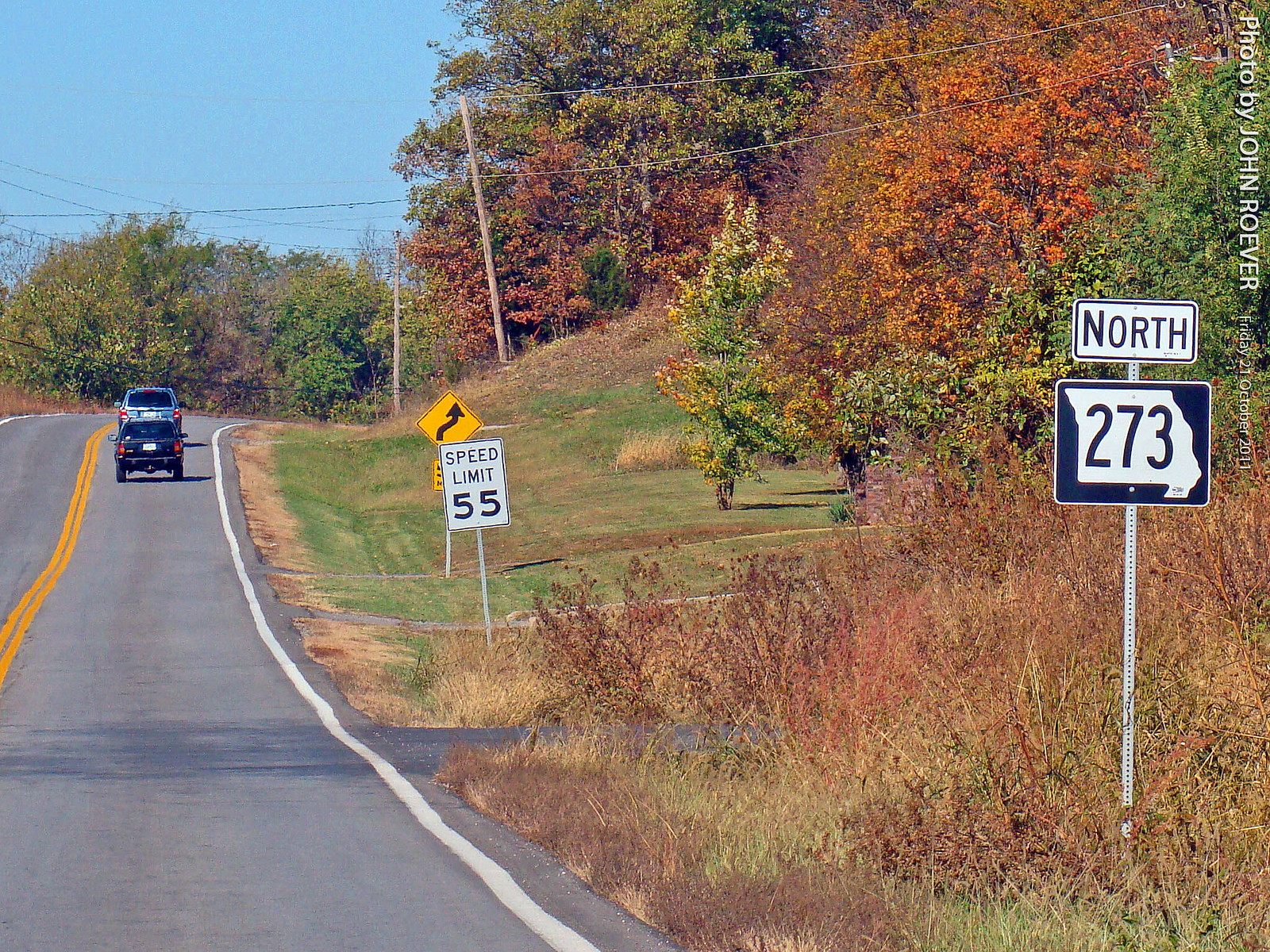This vibrant color photograph captures an inviting autumn roadside scene. On the left, a portion of a road is visible, extending toward the distance where two cars - one grey and one dark black - are seen driving away from the viewer. The surrounding landscape, framed by trees adorned in hues of golden orange and yellow, hints at the fall season in full swing. Above the trees, a network of power cables stretches against a backdrop of a clear blue sky.

In the background, more trees rise, adding depth to the image with their warm autumn foliage. Roadside signs punctuate the scene: prominently, a yellow sign with a curved black arrow and another white sign indicating a speed limit of 55 in black lettering. A grassy area beneath the trees transitions into a patch of overgrown orangey weeds closer to the road.

To the right, a sign directs travelers North along Route 273, with the number clearly printed in black on a white background. In the bottom left corner, a small, rotated text reads "Photo by John." Beneath this tribute, the name "Rover" appears, accompanied by smaller, unreadable text.